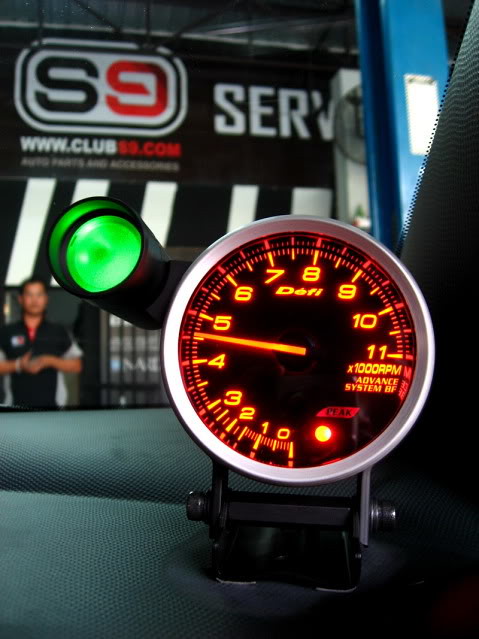In the photo, a black sign with diagonal white lines at the bottom stands prominently in the background. At the top of the sign is a rectangular shape with rounded edges, featuring a black 'S' and a red '9'. Below this, there is partially legible text, "www.clubsomethingisillegible.com." To the right of the main text are the letters "S-E-R-V." In the foreground, towards the left, a man faces the camera. He is wearing a black shirt with a gray stripe running down the side. To his left is an unidentified object composed of multiple gray rectangular shapes stacked vertically. In the immediate foreground, the dashboard of a car is visible, sporting a bluish-gray hue. Centrally located on the dashboard is an RPM gauge with a silver round border, a black center, and orange numbers ranging up to 11, indicating "X 1000 RPM." A green light is positioned at the upper left of the gauge.